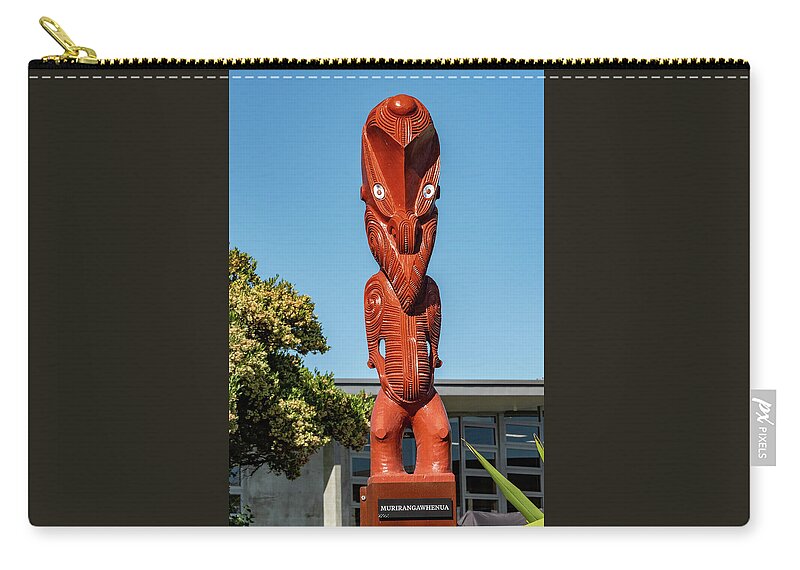This is a color photograph of a small black zippered pouch, resembling a change purse. It features a gold zipper along the top, starting on the left, and a tag on the side that reads "PX Pixels." Central to the pouch is a printed photograph of a striking wooden tribal sculpture with very exaggerated humanoid features. The sculpture, tinted red, has prominent and large white eyes, a protruding belly, and thick legs, all adorned with swirly tribal lines over the arms, face, and belly. The figure's detailed facial features include a large forehead, long jaw, and deep grooves for eye sockets. Surrounding the sculpture in the background of the photograph are a building and a tree on the left-hand side. The pouch is meticulously finished with white dotted stitching along the top, adding to its intricate design.